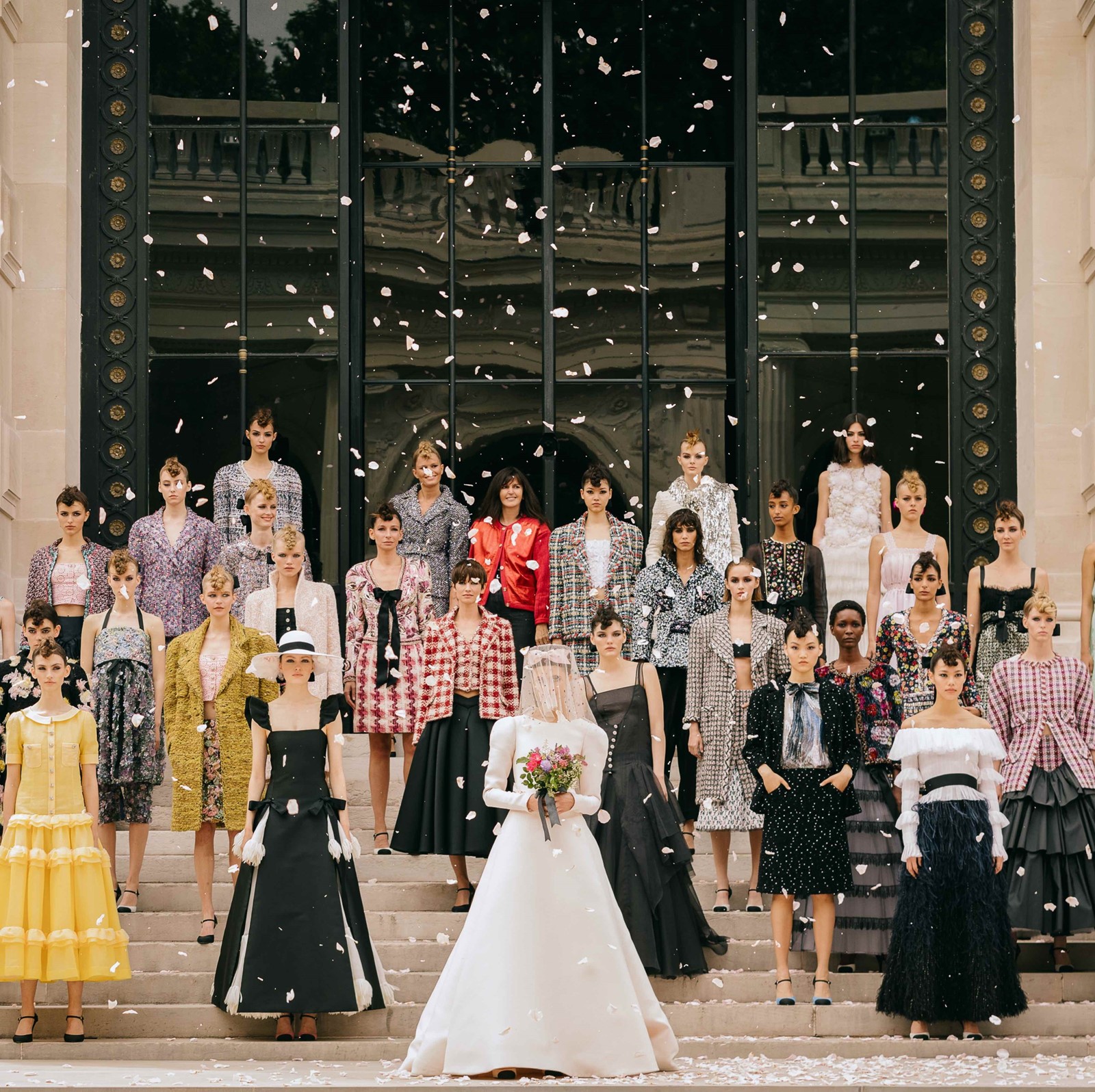In this photograph, a diverse group of individuals, including Caucasian men and women as well as a woman of color, are gathered on the steps of an imposing building. The background features sleek, dark-tinted windows that glint in the light, reflecting parts of the scene and enhancing the modern architectural feel. The majority of the women are elegantly dressed in long gowns, which are predominantly in black and white hues. Some have accessorized their outfits with long-sleeve jackets that drape over their dresses, adding sophistication to their ensemble. Several of the women are adorned with decorative hats, featuring floral embellishments, which add a touch of classic elegance to the scene. Among them, one woman stands out, holding a bouquet of roses; she appears to be a bride, donned in a traditional white wedding gown complete with a veil that delicately covers her face. The composition captures a moment of post-ceremony joy and celebration.